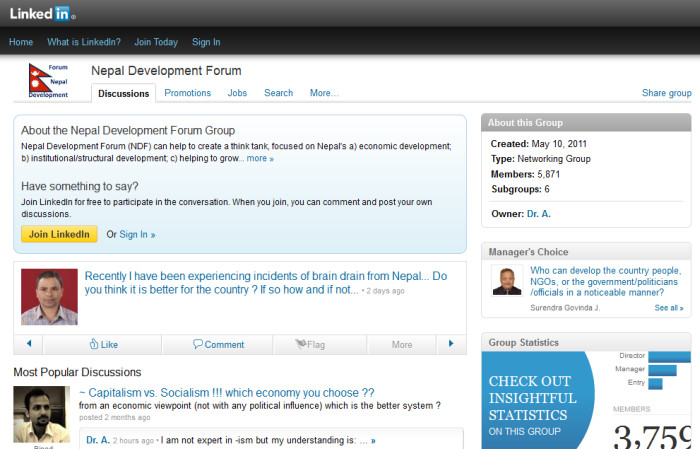The image depicts a LinkedIn webpage with a layout approximately 30 to 50% wider than it is tall. The topmost section features a dark gray horizontal bar, prominently displaying the LinkedIn logo in the upper left corner. Below this, there is a black navigation bar with light blue text, listing menu options: Home, What is LinkedIn?, Join Today, and Sign In.

The main content area of the webpage transitions to a white background. In the upper left corner, there is a red flag icon pointing to the right, labeled "Forum Nepal Development." Adjacent to this icon, the title "Nepal Development Forum" is displayed, followed by a row of navigation tabs: Discussions (selected), Promotions, Jobs, Search, and More, with Promotions highlighted in blue.

On the left side of the content, there is a section with a light blue background titled "About the Nepal Development Forum group." Below this heading, several paragraphs of descriptive text provide information about the group.